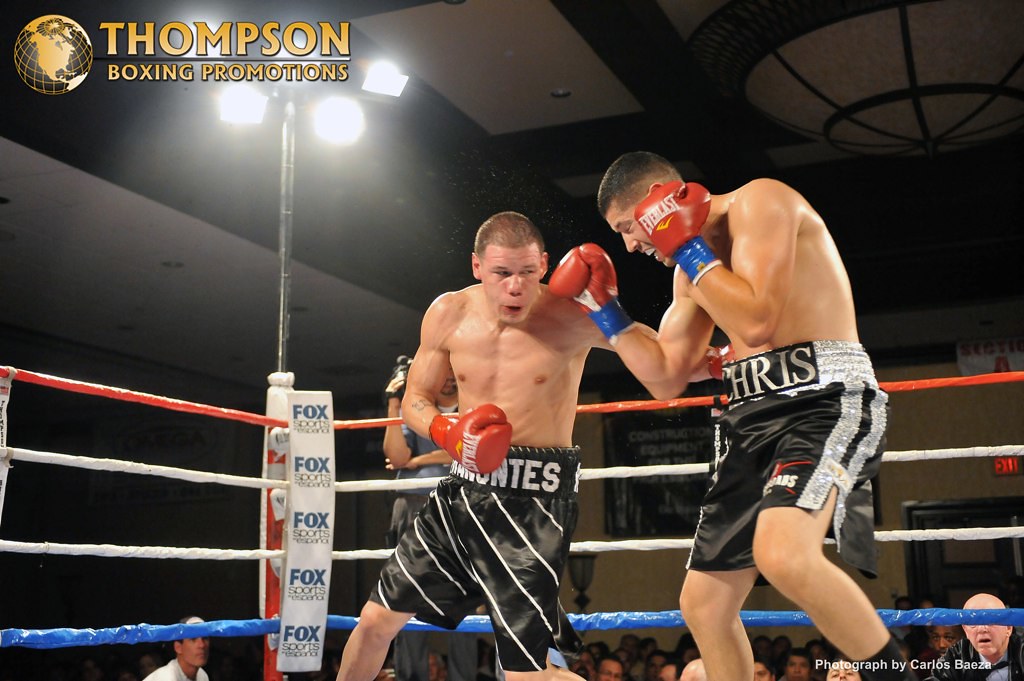The photograph captures an intense live boxing match between two muscular Caucasian men. Both boxers are wearing black shorts, with one athlete sporting white diagonal stripes on his trunks and a belt partly displaying the name "Montez." The other boxer dons black-and-white shorts with a silver sparkle stripe and a belt showing the name "Chris." Both fighters are donning red boxing gloves with the "Everlast" logo in white. The scene is set in a ring with red, white, and blue ropes. The ring's corner prominently features a white flag with "Fox Sports" in bold blue lettering, and a top banner highlighting "Thompson Boxing Promotions" alongside a gold wireframe globe. Bright lighting fixtures hang above, illuminating the fighters, who are visibly tired and sweaty, locked in the heat of the battle. One boxer appears poised to strike, while the other exhibits an expression of potential pain, vividly conveying the dynamic and vigorous nature of the moment.